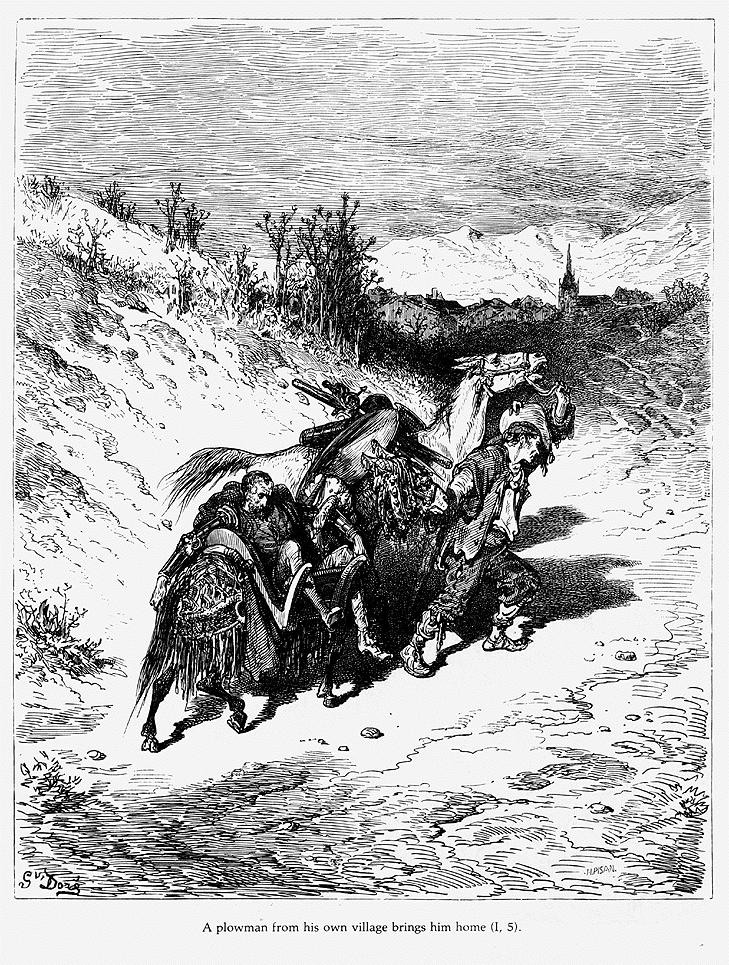This is a detailed black and white pen and ink drawing depicting a plowman from his village bringing an injured person home. The scene shows a rugged landscape with the group traveling through a valley between hills that rise about 10 to 20 feet. At the bottom of the image, there's text reading "A plowman from his own village brings him home (1,5)." The drawing focuses on a man leading a horse up a hill. The horse, which appears to be burdened with a saddle and various items, is being guided by the plowman who also seems to have hold of a donkey. 

The donkey carries an older man dressed in a coat of arms but without his helmet. Surrounding the group are rough grounds with mountains looming in the background and a church steeple visible in the distance, suggesting they are approaching a village. The composition is vertically oriented, with a wider border at the bottom framing the descriptive footer. The image conveys a sense of struggle and perseverance, reminiscent of scenes from Don Quixote as an injured master is brought back to safety, emphasizing the effort and care involved in their journey home.